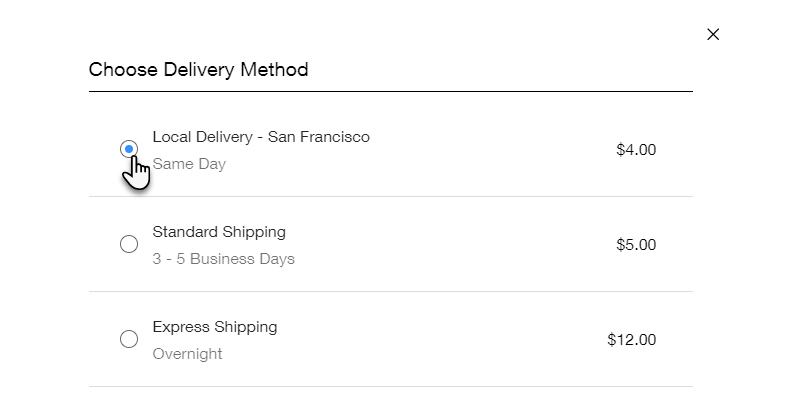In this image, we see a screenshot from what appears to be an online purchase interface. The screenshot prominently features a section where the user is prompted to "Choose Delivery Method," as indicated by the text in the top left corner. In the upper right corner, an 'X' button is positioned, presumably to exit the selection screen.

Below the instructional text on the left, there is a black horizontal line, under which three delivery options are clearly delineated. The first option is "Local Delivery - San Francisco Same Day for $4," clearly marked as selected. This is indicated by the blue filled-in circle next to the option, along with a mouse cursor hovering over it.

The second option is "Standard Shipping - 3 to 5 Business Days for $5." This choice is represented by an unfilled gray circle, showing it is not currently selected. 

The third and final option listed is "Express Shipping - Overnight for $12," also indicated by an unfilled gray circle, suggesting this option is likewise not chosen. 

Thin gray lines separate each delivery option, providing a visual distinction between the various choices available to the user.